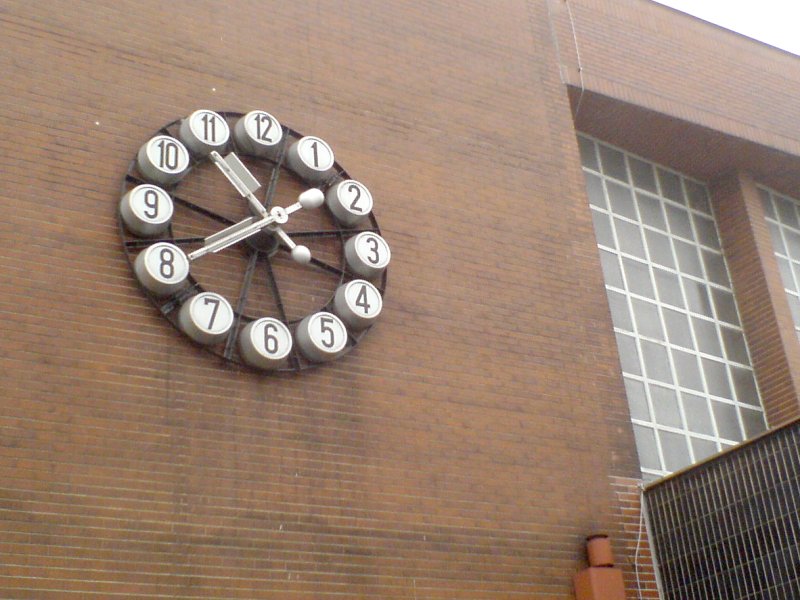Here is a cleaned-up and detailed caption for the image described:

"In this color photograph, we see a clock affixed to an exterior wall made of small red bricks. The clock features a design reminiscent of a wheel, with dark metallic spokes extending from its center. Surrounding the wheel are circular markers for the numbers, each with a dark grey edge and a white face, displaying black numerals from 1 to 12. The clock’s hands are white, but their precise positions are difficult to discern; the longer hand points between the 8 and 11, while the shorter hand points between the 2 and 4. These hands also have small round protrusions near their ends.

To the right of the clock, several large windows with square glass panes and white rims can be seen. At the bottom of the image, a dark fence runs along the lower edge of the building. Below this fence, there are several wooden shapes, including a square piece on top of a larger square, and a rectangular piece positioned to the right. These wooden elements form an outline that vaguely resembles a human figure, although it appears abstract and could be AI-generated or a character from a game."